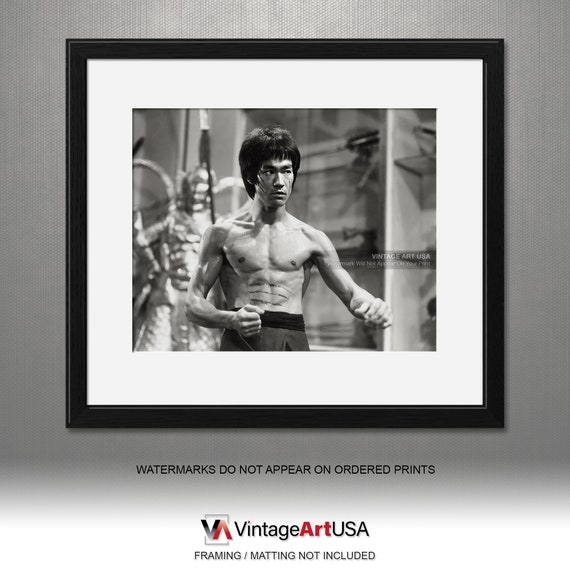This promotional webpage features a black and white poster of Bruce Lee, showcased within a sleek black frame from Vintage Art USA. The image, likely a still from one of his iconic movies, captures Bruce Lee shirtless and in his classic karate fighting stance. He wears athletic-style pants and gazes fiercely off-camera to the right. His iconic haircut and a claw slash across his midsection are prominently visible, marking his intense presence. The background fades into a blur, showcasing what appears to be a golden statue and various martial arts weapons, keeping the focus sharply on Bruce Lee in the foreground. The frame does not include matting, and while the displayed picture carries the Vintage Art USA logo, ordered prints are free from watermarks. Vintage Art USA also offers custom framing services for any photo you choose to send them.